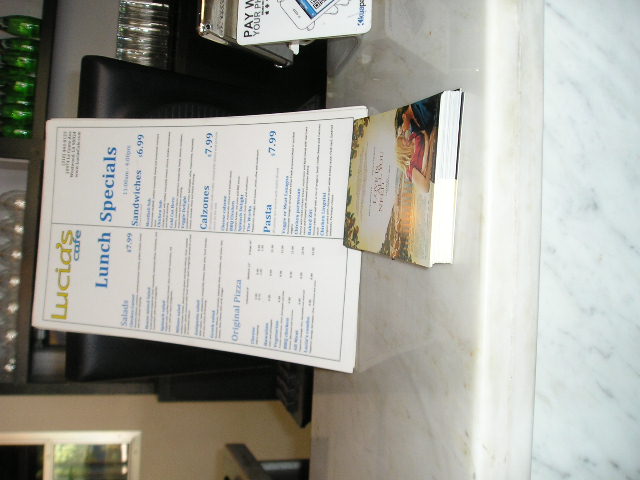The image depicts an inviting restaurant scene framed in a sideways orientation. Dominating the foreground is a dual-layered countertop. The bottom layer is a striking marbled granite with elegant white, gray, and tan streaks, while the top layer features a more muted brown, beige, and off-white surface, where various items rest. In the background, a window reveals an exterior view adorned with a green tree bathed in daylight, casting a soft natural glow into the scene. 

Against the window stands a multi-tiered brown shelf. The top shelf holds an orderly row of clear wine glasses, while the middle shelf showcases green wine glasses, adding a touch of color and sophistication. The bottom shelf is stocked with standard clear drinking glasses.

On the countertop, a sign reads, "Pay with your phone," emphasizing the restaurant's modern conveniences. Next to it, a "Lucia's Cafe Lunch Specials" menu is propped against the back of a black computer screen, likely capturing the daily culinary delights offered at this charming establishment.